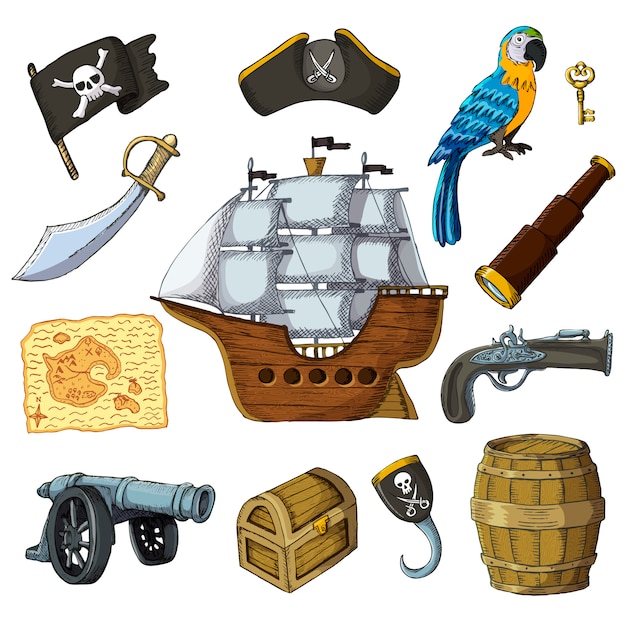The image contains a vibrant collection of cartoon drawings, all themed around pirates and scattered across the canvas. In the top left, a black flag featuring a white skull and crossbones flutters from a brown stick. To the right, a black tricorn hat trimmed in gold boasts two crossed white swords on its front. Next to the hat, a colorful parrot with blue feathers on its back, a yellow belly, and a green spot atop its head perches confidently. Further right, an old-fashioned gold key gleams. 

In the second row, a curved scimitar with a gold hand protector starts the lineup, followed by a tan and yellow map of an island. Adjacent to the map, a sturdy brown cartoon boat with large white sails anchors the pirate theme. Scattered around these central objects are additional pirate essentials such as a wooden barrel, a treasure chest, a telescope, a revolver, and a cannon. Together, these lively illustrations evoke a playful pirates' adventure on the high seas.